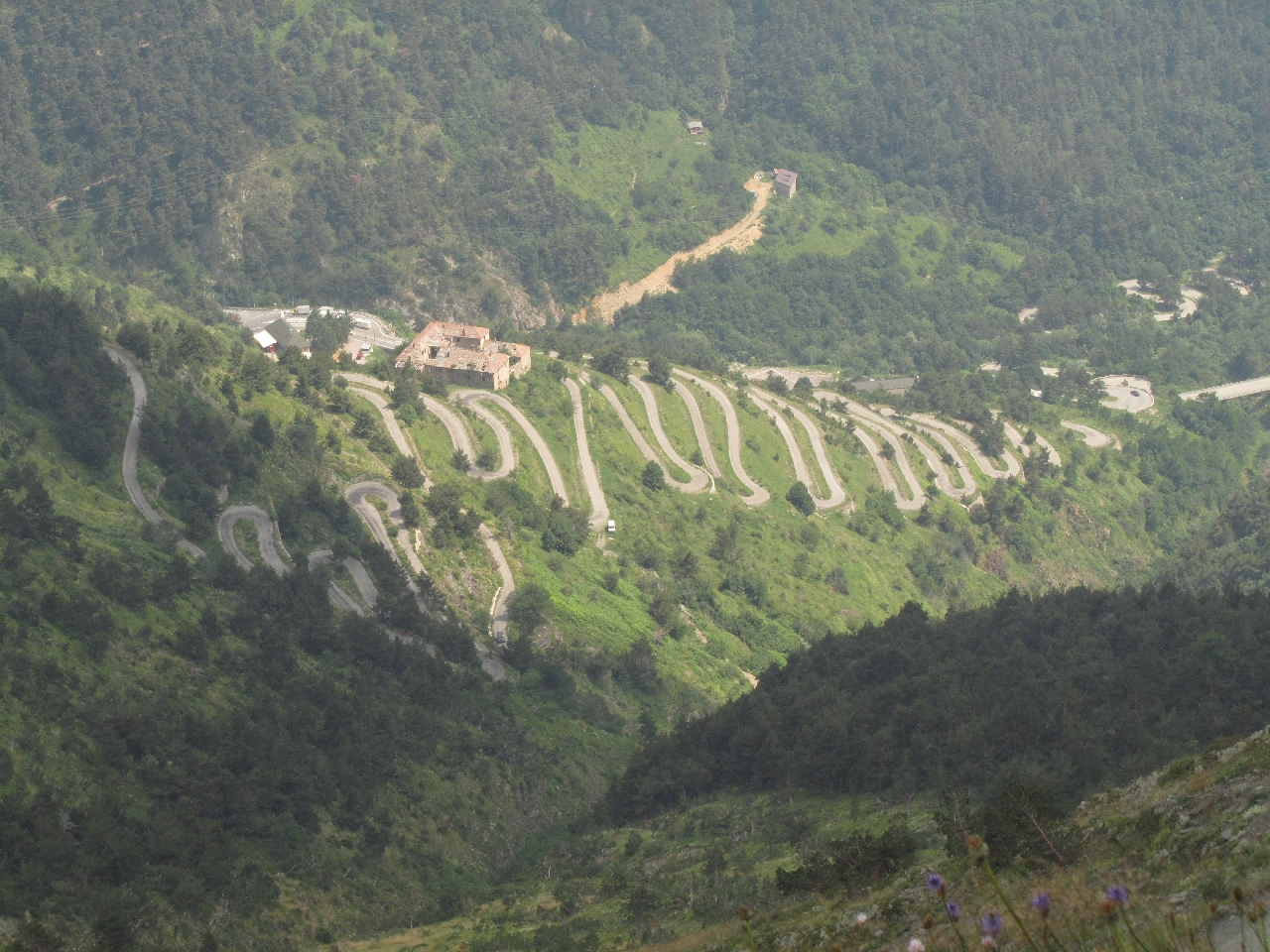This colored aerial photograph, slightly overexposed and enveloped in mist, captures a vast valley with a prominent winding dirt road that zigzags up and down the mountain in loop formations. The twisty road, resembling a racetrack, spans across the center of the image from left to right, moving back into the mountains. The scene is filled with lush green trees and abundant greenery across the foothills and valley, creating a sense of dense foliage. In the foreground, towards the bottom right, small purple flowers are visible, adding a delicate touch of color. Near the top of the hill, partially hidden by trees, a structure resembling a house or building is seen, potentially with a parking lot or vehicles nearby. Despite the misty, overcast ambiance with grayish-green hues, patches of sunlight cast shadows across the scenery, enhancing the photograph's depth and texture.